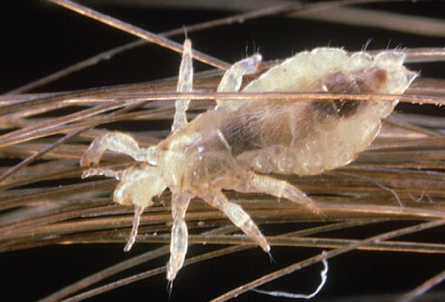This is a color photograph in landscape orientation, presenting an extreme close-up microscopic view of a head louse. The insect, approximately one centimeter in length, displays a translucent body through which its internal organs are partially visible in dark and light brown shades. The head, pointed to the bottom left, is yellow and translucent with two antennae extending outward. The louse's elliptical body has a square middle section that rounds towards the back. It possesses six translucent legs, each with black extensions resembling fingernails. The insect is perched on several orange strands of hair, with one hair strand arching over its body. The dark background accentuates the detailed, photographic realism of the image, creating a stark contrast that highlights the intricate features of this nefarious-looking creature.